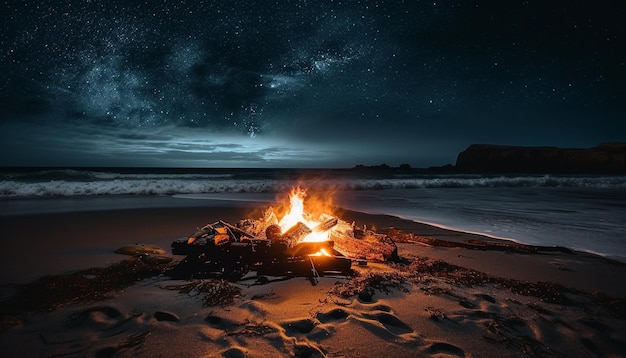The image captures a serene beach scene under a clear starry night. Dominating the foreground is a glowing campfire with logs stacked around it, casting a warm light onto the sandy beach. Footprints are visible in the sand, evidence of previous visitors. Just beyond the fire, waves crash gently onto the shore, their white crests distinct against the dark ocean. To the right, a rocky cliff silhouette rises, adding a dramatic element to the scene. The sky above transitions from a deep blue near the horizon to almost black, dotted with countless stars, and even hints at faint galaxies with vibrant patterns. This realistic photograph beautifully combines elements of earth, water, fire, and sky, creating an enchanting nighttime beachscape.